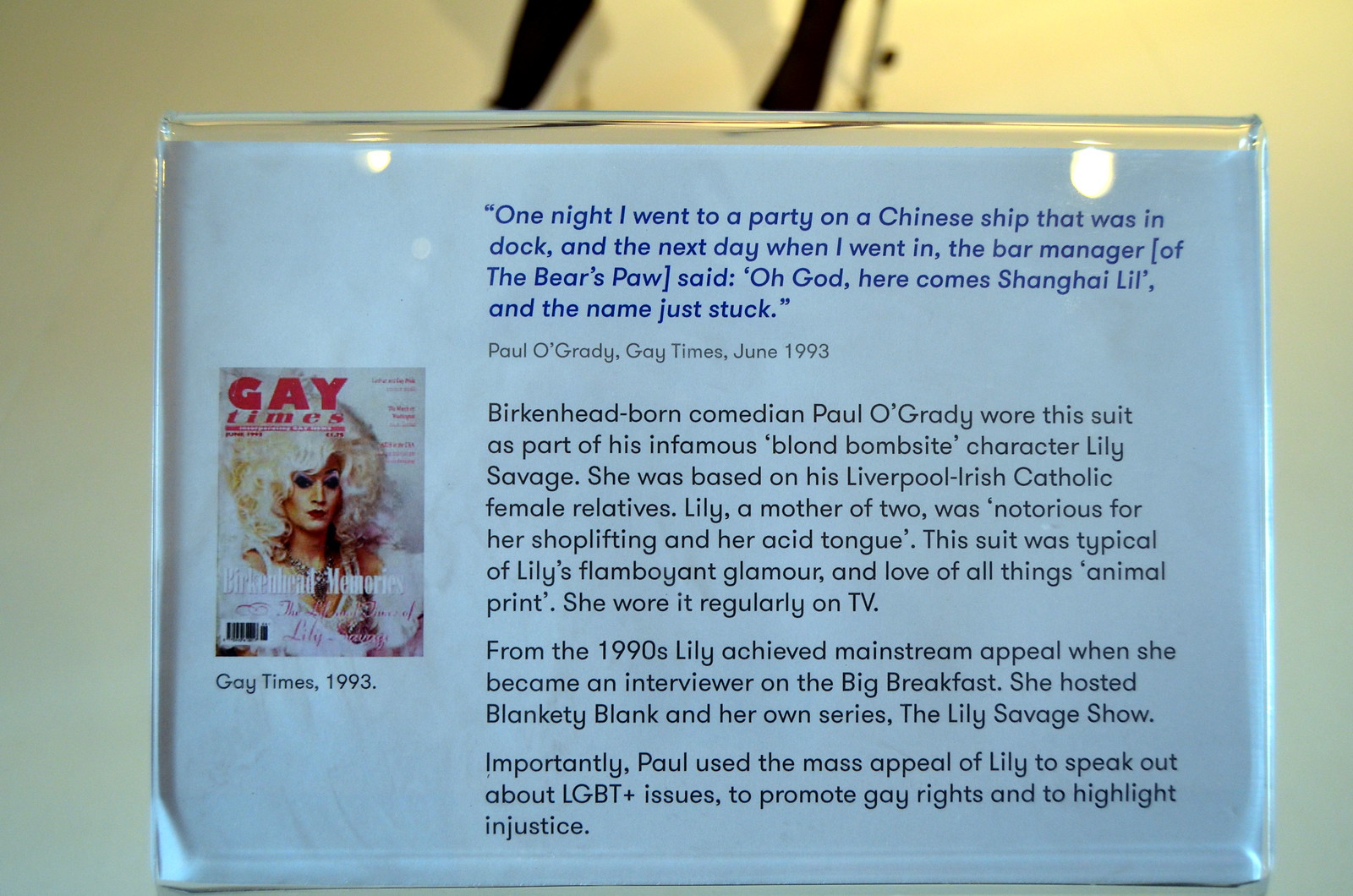This image displays a white piece of paper encased in a plastic covering, featuring blue and black text. In the left-hand corner, there’s a cover of a magazine named "Gay Times" in red letters, depicting Paul O’Grady’s drag persona, Lily Savage, characterized by a voluminous white wig. The blue text atop reads: “One night I went to a party on a Chinese ship that was in the dock, and the next day when I went in, the bar manager said, ‘Oh God, here comes Shanghai Lil,’ and the name just stuck. Paul O’Grady, Gay Times, June 1993." Further down in black text, it details Lily Savage as a creation of Birkenhead-born comedian Paul O'Grady, inspired by his Liverpool Irish Catholic female relatives. Lily, a notorious figure for her shoplifting and sharp wit, became a celebrated character, regularly appearing on TV in flamboyant, glamorous suits often featuring animal prints. From the 1990s, Lily Savage achieved mainstream success, featuring on shows such as "The Big Breakfast," hosting "Blankety Blank" and her own series, "The Lily Savage Show." Paul O’Grady leveraged Lily’s popularity to advocate for LGBT+ issues and promote gay rights.